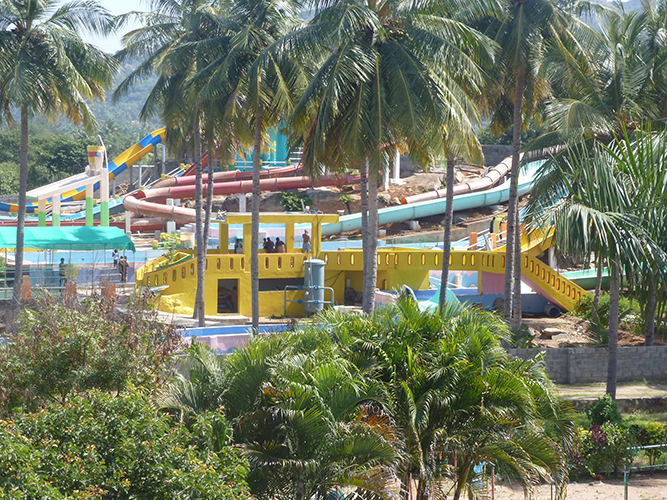The image showcases a vibrant water park under a sunny sky, with a variety of colorful water slides and a lush backdrop of trees. Dominating the foreground are tall palm trees, approximately nine in number, standing before a concrete block wall and lush green shrubbery. Beyond this green barrier, a bustling array of water slides can be seen: a striking yellow and blue striped slide that twists down into a green pool, a nearby red enclosed tube slide, and an open blue slide. Adjacent to these slides is a distinctive yellow platform resembling a fish, with its 'tail' extending long to the right and forming a V shape. Seven people are seen standing on part of this platform, though their activities are unclear. Adding to the greenery, a row of tall pine trees frames the back of the image, with shorter pine trees interspersed in the front. Additional park features include tents where people, likely waiting for their turn on the slides, are gathered. The entire setting is bathed in sunlight, emphasizing the hot and cheerful atmosphere of the water park.